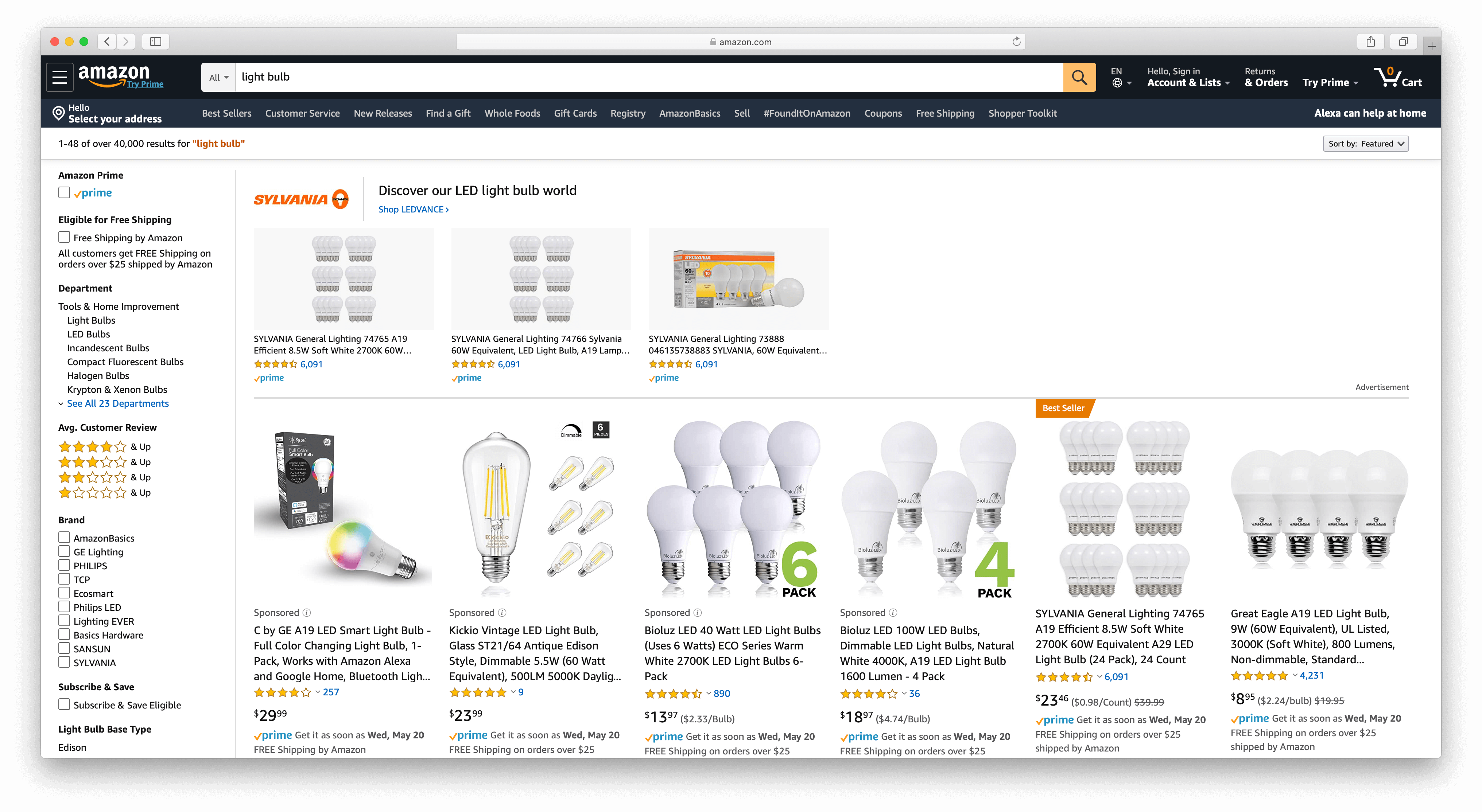The image displays an Amazon search results page with the term "lightbulb" entered in the search bar. At the top of the search results, there is a banner featuring the Sylvania logo and the tagline "Discover our LED lightbulb world." Directly beneath the banner are three featured products:

1. On the left is the "Sylvania General Lighting 74765A19 Efficient SW Soft White 2700K 60 Watt" LED light bulb, which has received a rating of four stars based on approximately 6,961 reviews, though the exact number is slightly blurry.
   
2. In the center is the "Sylvania General Lighting 74765 Sylvania 60 Watt Equivalent LED Light Bulb," boasting a rating of about four and a half stars.

3. On the right is the "Sylvania Lighting 73888 60 Watt" LED light bulb.

Below these featured items is a different section of search results displaying six additional lightbulb options arranged in a horizontal row, each accompanied by a logo.